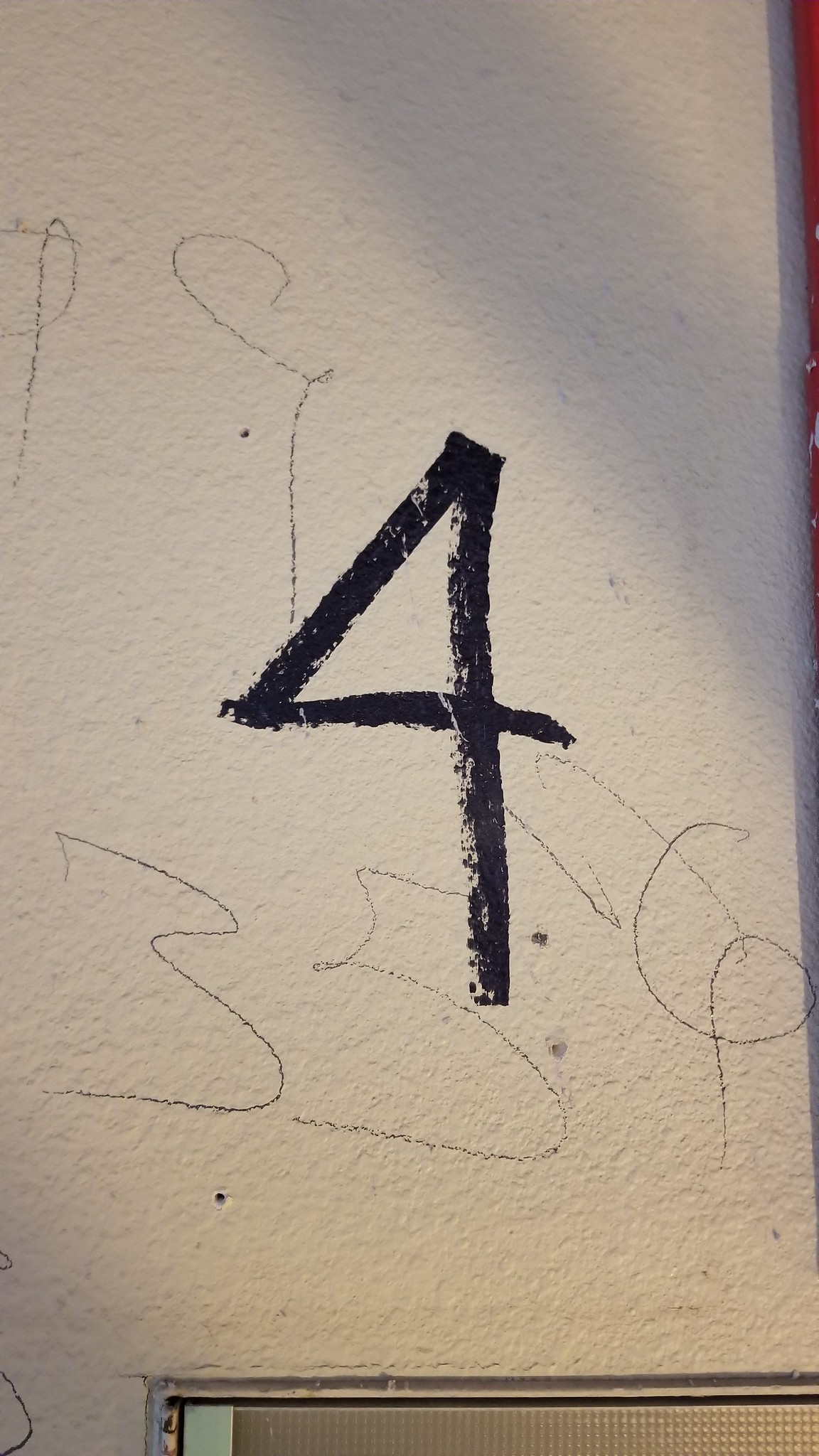The image depicts a white stucco wall inside a house, potentially above a metal-framed doorway or window. A rectangular shadow stretches across the wall towards the upper right, adding a touch of depth to the scene. Dominating the center of the wall is a bold number "4" drawn in black marker, in a European style with no open top, which stands out prominently against the textured backdrop. Above the "4" is an incomplete numeral "9", drawn possibly in crayon. Below the "4", the number "3" appears slightly to the left, and directly underneath, a number "5". To the right of the "5", there's a number "6" with two lines extending from it, resembling an "11". The wall also bears several faint and indeterminate scribbles, likely made with a quick pencil or pen, imparting a sense of casual creativity to the setting.